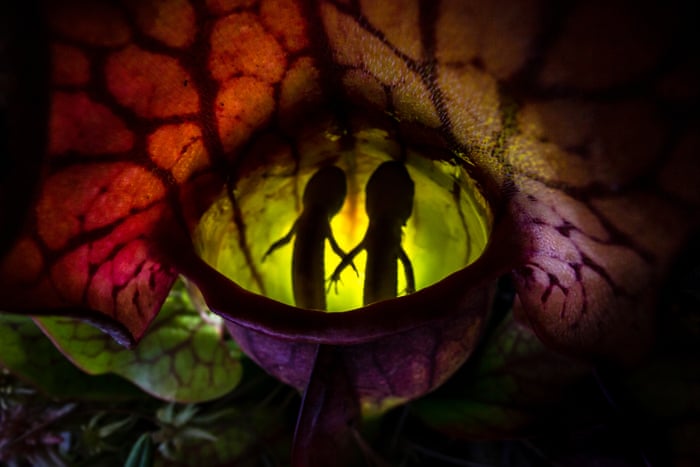This abstract and intriguing image features a central purple bowl with a bright green interior, set against a backdrop of dark leafy shrubs. The bowl appears to contain two enigmatic, black silhouetted forms with what look like elongated arms or pistils, resembling shadowy figures. Surrounding this central element, vibrant hues of red, orange, and purple blend with the green leaves at the bottom of the image. The upper part of the photograph showcases colorful leaves—possibly butterfly wings—displaying shades of purple, red, and orange with visible veins. The scene is bathed in varied lighting, with a yellow glow at the center, transitioning to purples on the right, reds on the left, and browns on the top right. The absence of any identifying information, humans, animals, text, or annotations adds to the captivating mystery, making this image a complex blend of natural and abstract elements.